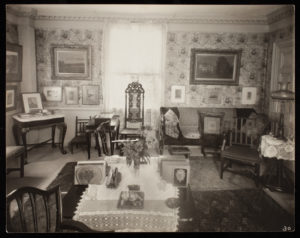The photograph depicts a low-resolution, black and white image of a living room or parlor with a distinct Victorian ambiance. Central to the room is a table draped in a light-colored tablecloth, possibly white, flanked by various high-backed, ornate wooden chairs, suggesting tufted seats. The arrangement of the furniture lacks clear organization, with chairs surrounding the table but blocking part of a wooden sofa adorned with a light-colored cushion. To the left, a high desk with a light top can be seen, along with additional tables and seating scattered throughout. The walls are adorned with an array of paintings and picture frames, some positioned next to a window covered by a sheer curtain. A small coffee table with a doily-style table runner is placed in the foreground, complemented by throw rugs beneath. The wallpaper appears to have a busy, possibly floral pattern, adding to the intricate, old-timey aesthetic of the space. Additionally, subtle gas lighting fixtures are visible on the right wall, enhancing the room’s vintage charm.